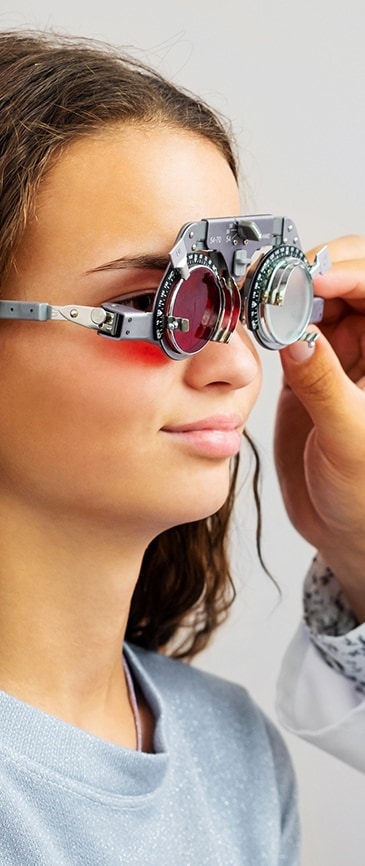In this detailed image, a young woman with long, wavy brown hair flowing past her shoulders is having her vision checked. She is wearing a light gray sweatshirt paired with a thin, light-colored necklace. The woman, who appears to be a white woman with a slight tan, is smiling subtly, looking towards the right side of the picture. A complex optometric device with various dials and tiny numbers is held in front of her eyes. The lens on her left side is white, while the lens on her right side is red. The lenses are being adjusted by a person's hand, which is visible in the frame. This person, likely a doctor, is identifiable by the white lab coat they are wearing over a patterned long-sleeve shirt. The doctor's hand is shown pinching the device on the left side, adjusting it precisely. The close-up view captures the woman from the top of her head down to about her chest area, showcasing her engaged expression and the specialized equipment being used in the eye examination.